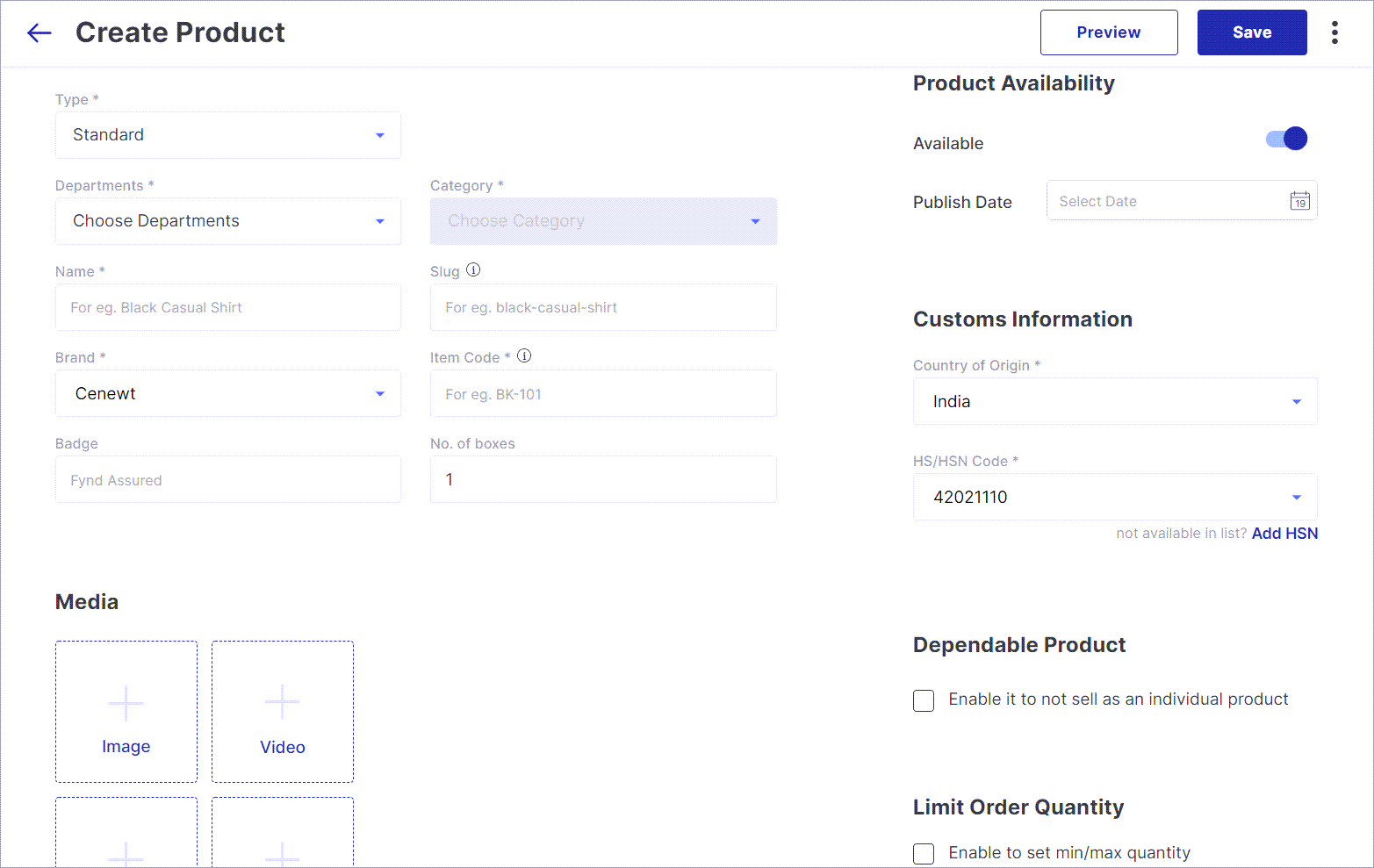The image features a user interface for creating a product listing. Encased in a white box with a gray border, the top left corner displays a blue arrow pointing left. Adjacent to this arrow, black bold letters spell out "Create Product."

On the far right side, there is a white rectangle with the word "Preview" in blue, followed by a blue rectangle labeled "Save" in white text. Above these, three vertically-stacked black dots provide additional options.

On the left side of the interface, several fields are available for user input. The "Type" field has a dropdown menu currently set to "Standard." Below this, a "Department" dropdown menu reads "Shoe Department." The subsequent "Name" field is a text box where users can enter the product name.

Underneath, a "Brand" field, accompanied by a dropdown menu, features a currently blurry and small-text selection, likely reading "CNEWT." The "Badge" field below contains an area for typing, with "Find Assurance" pre-entered.

At the lower section, bold black letters indicate "Media," with clickable options to add both videos and images.